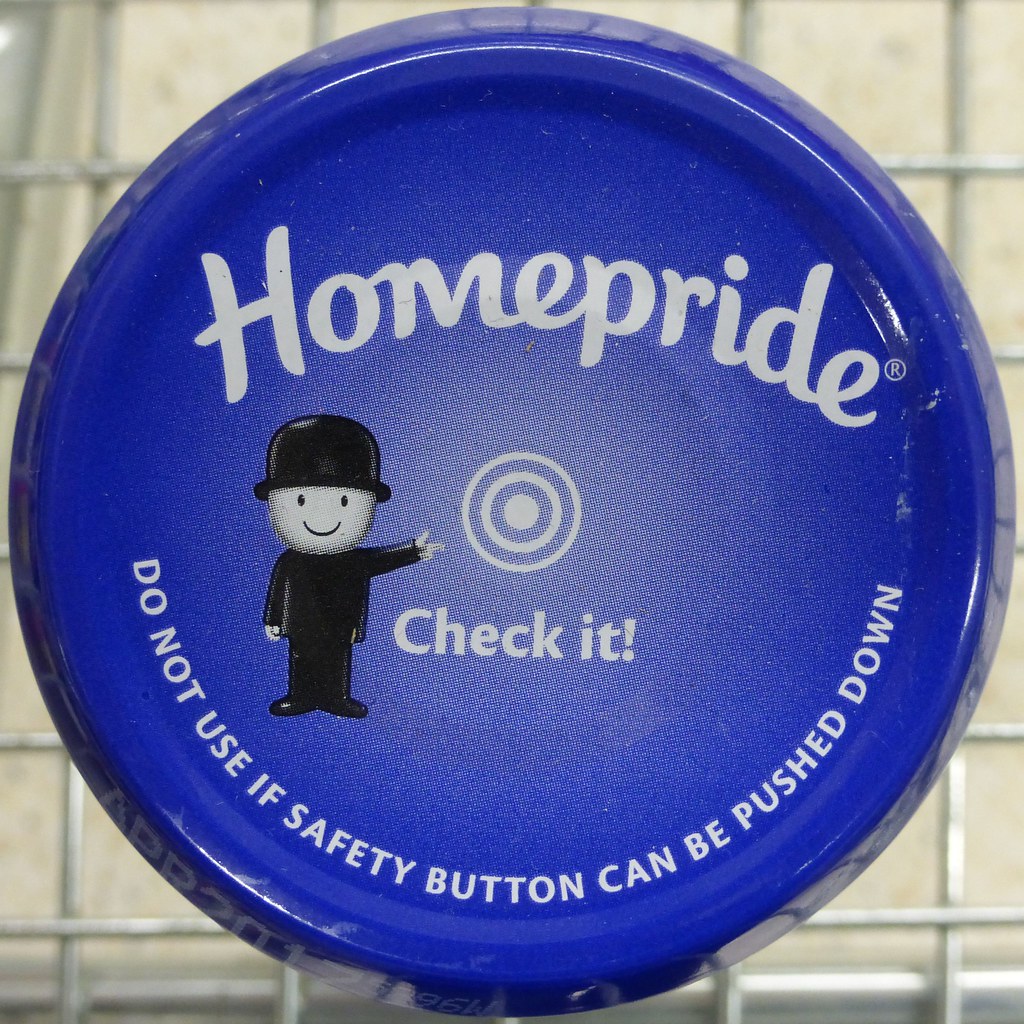This image features a blue, round bottle cap prominently designed and marked with the brand "HOME PRIDE" in bold white letters at the top. Below the text, there is a distinctive cartoon character—a man with a derby hat, dressed in a black outfit with a white face—pointing towards the center of the cap. This center area contains a white, round button with concentric circles and the words "CHECK IT" inscribed. At the bottom edge of the cap, a safety warning is displayed in a semi-circular arrangement: "DO NOT USE IF SAFETY BUTTON CAN BE PUSHED DOWN." The bottle cap appears slightly dirty and is situated on what resembles an aluminum grate, possibly part of a dish drainer or a table surface. The background of the image includes elements that look like a metal fence. The visual design and the directional gesture of the cartoon character emphasize the importance of checking the safety button.